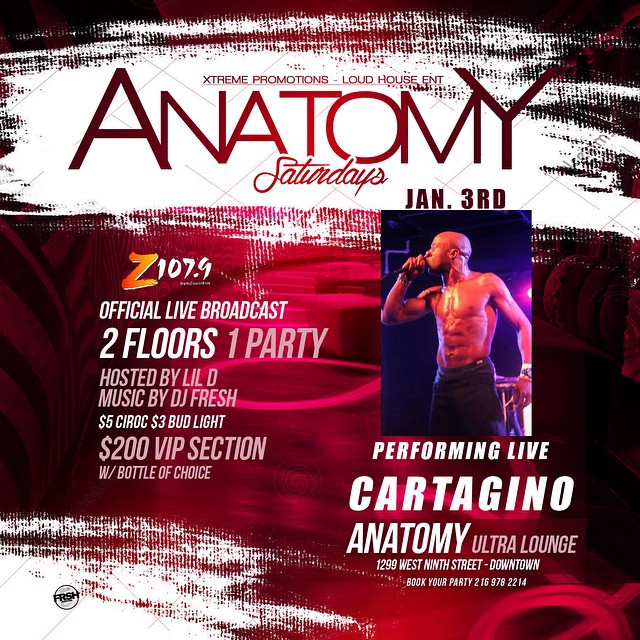This is a highly detailed poster advertising Anatomy Saturdays, a lively club party happening on January 3rd. The event is promoted by Extreme Promotions and Loud House Entertainment, and it prominently features a shirtless man, Cartangino, passionately singing into a microphone. The performance is highlighted with the phrase "Performing Live" in white text next to his image. The event promises an official live broadcast spanning two floors, transforming into one massive party. Hosting duties are managed by Lil D, with music by DJ Fresh setting the vibe. The poster also showcases enticing deals, including $5 CIROC, $3 Bud Lights, and a $200 VIP section with a bottle of choice. This vibrant event is set to take place at Anatomy Ultra Lounge, located at 1299 West 9th Street, Downtown. For bookings, the contact number provided is 216-978-2214. The background of the poster is a dynamic reddish-pink with abstract swathes of white adding to the excitement.